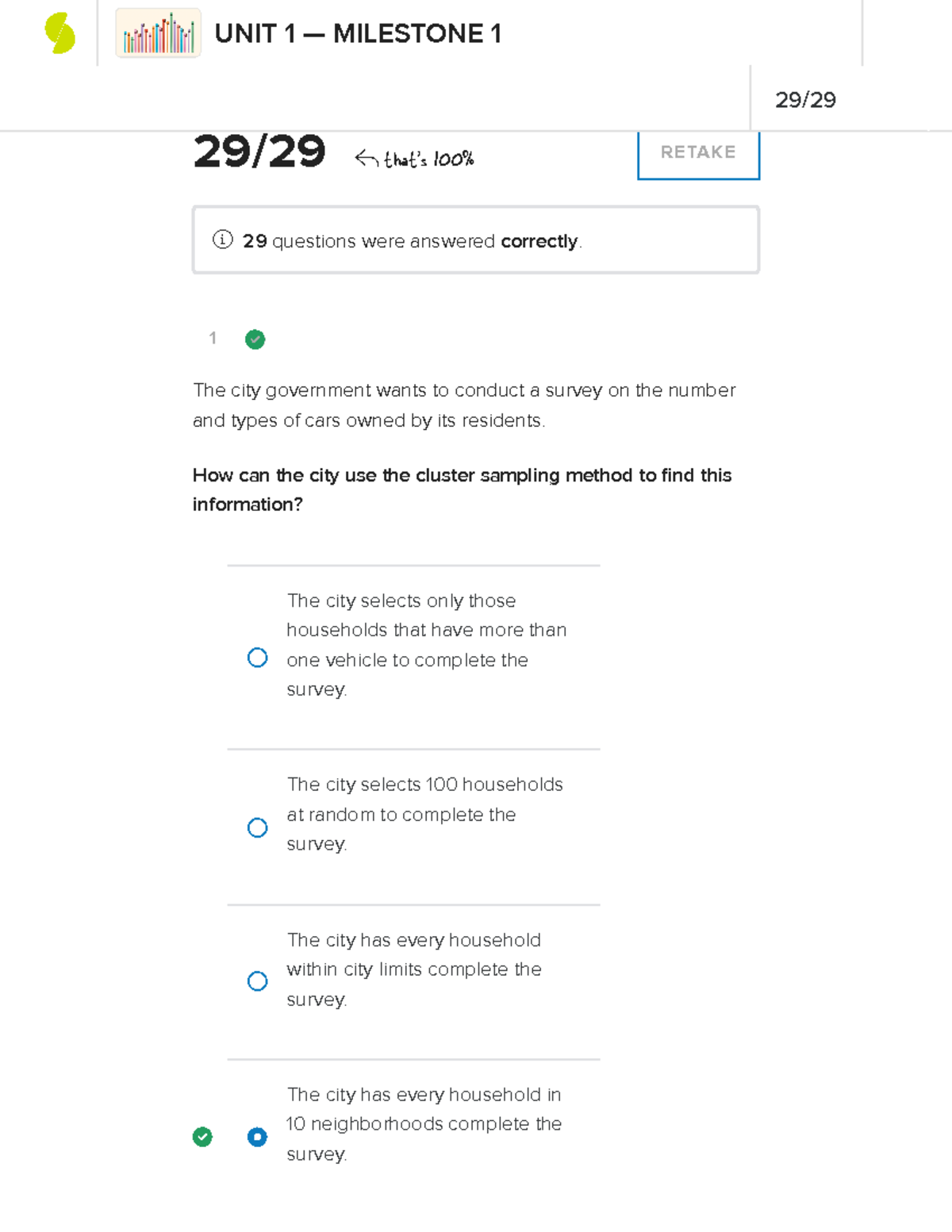This image appears to be a screenshot of a test question from an assessment named "Unit1-Milestone1," as labeled at the top of the page. To the left of this title, there is a bar graph, though its specific details are indiscernible. The test seems to have been aced, as indicated by the score "29 out of 29," marked below the title, along with a handwritten note saying "100%." This note is placed within a white box outlined in gray, emphasizing the perfect score. Below this, the first question of the test is displayed, labeled as "1." The question reads, "The city government wants to conduct a survey on the number and types of cars owned by its residents. How can the city use the cluster sampling method to find this information?" Four answer choices are provided, and the respondent has correctly selected, "The city has every household in 10 neighborhoods complete the survey." This choice is indicated as the correct answer among the four options.